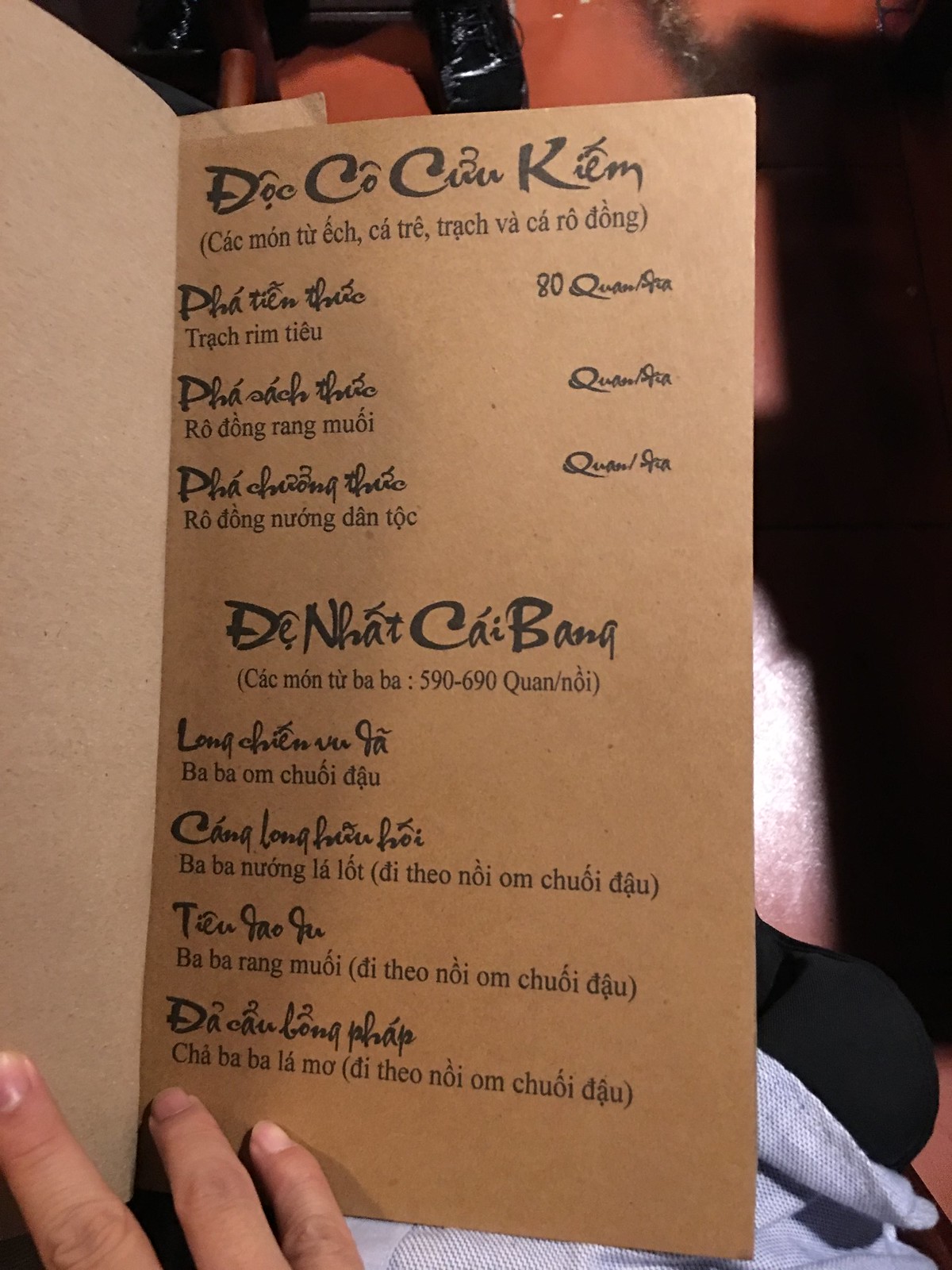In a portrait-oriented photograph, a person is seen holding open what appears to be a folded menu or program, written in an unfamiliar language. The document has an elegant, swirly title at the top, possibly reading "Dokko Kukiem." Despite potential French influences in the text, the language remains unidentifiable. The script includes a list of items with only one identifiable number, “80,” next to an entry. The content is printed on a brown piece of paper, which looks aged and slightly folded. The individual's hands, visible in the image, are gently spreading the paper to reveal its contents, suggesting it rests on their lap. The faint outline of their shirt is discernible at the bottom, adding to the casual, intimate setting. The overall ambiance of the photograph hints at an old-fashioned, possibly cultural document being examined with curiosity.